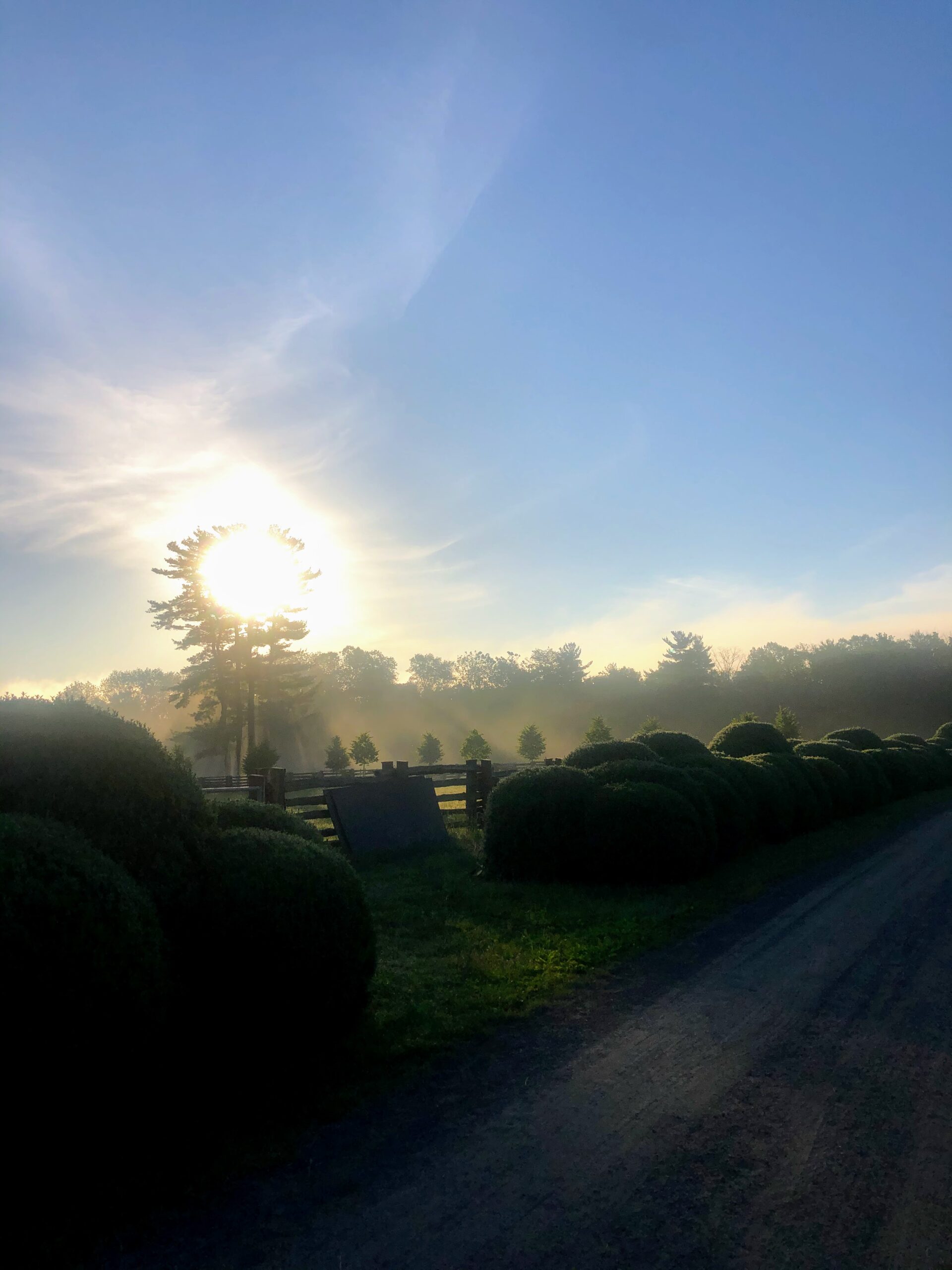The image depicts a serene country scene, captured from a Street View perspective. On the right side of the frame, a gravel road is partially visible, while to the left, an array of meticulously trimmed, bubble-shaped shrubs lines a small grassy pathway that leads up to a wooden fence. Leaning against this fence is a square object, possibly a board or a small billboard. The landscape extends into a field dotted with evenly spaced small trees, which gradually give way to a denser forest in the background. The sky occupies the upper half of the image, boasting a deep blue hue with several white streaks. The sun, positioned off in the distance, appears to be setting behind a tall tree, casting a warm glow through its branches and adding a sense of tranquility to the scene.